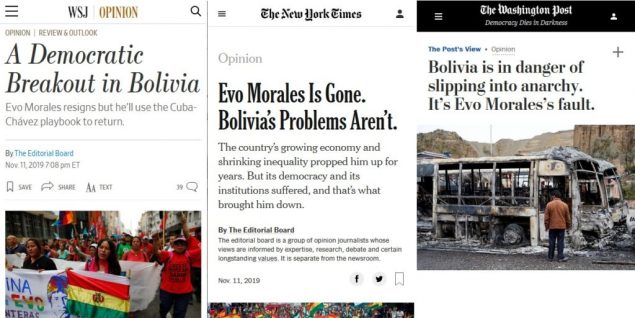**Description of the Image:**

This is a comprehensive screenshot displaying a webpage from The Wall Street Journal, showcasing three side-by-side opinion articles from different major newspapers: The Wall Street Journal, The New York Times, and The Washington Post. Each article discusses the political situation in Bolivia following Evo Morales' resignation on November 11, 2019.

1. **The Wall Street Journal**
   - **Category:** WSJ / Opinion
   - **Title:** "A Democratic Breakout in Bolivia"
   - **Subtitle:** "Evo Morales resigns, but he'll use the Cuba Chavez playbook to return."
   - **Byline:** The Editorial Board
   - **Date and Time:** November 11, 2019, 7:08 p.m. Eastern Time
   - **Engagement Icons:** Options to save, share, and interact with the text.
   - **Reader Interaction:** Shared or liked by 39 users.
   - **Image:** The accompanying image shows a protest scene. People are demonstrating on a street, with one individual in the forefront holding a flag with horizontal orange, yellow, and green bars. Partially visible beside the flag is a man's face accompanied by some partially obscured text to the left of it.

2. **The New York Times**
   - **Category:** Opinion
   - **Title:** "Evo Morales is Gone. Bolivia's Problems Aren't."
   - **Subtitle:** "The country's growing economy and shrinking inequality propped him up for years, but its democracy and its institutions suffered. And that's what brought him down."
   - **Byline:** The Editorial Board, a group of opinion journalists whose views are informed through expertise, research, debate, and long-standing values, distinct from the newsroom.
   - **Date:** November 11, 2019
   - **Image:** The top of what appears to be the same protest scene depicted in The Wall Street Journal image, suggesting a larger crowd context.

3. **The Washington Post**
   - **Category:** Opinion (The Post's View)
   - **Motto:** "Democracy Dies in Darkness"
   - **Title:** "Bolivia is in Danger of Slipping into Anarchy. It's Evo Morales' Fault."
   - **Image:** The image features a burnt bus, showing only its metal framework left intact. A man stands in front of this bus, set against a backdrop of beige, rocky mountains.

Each article provides a unique perspective on the Bolivian political crisis, augmented by striking images that depict the unrest and chaos following Morales' resignation.